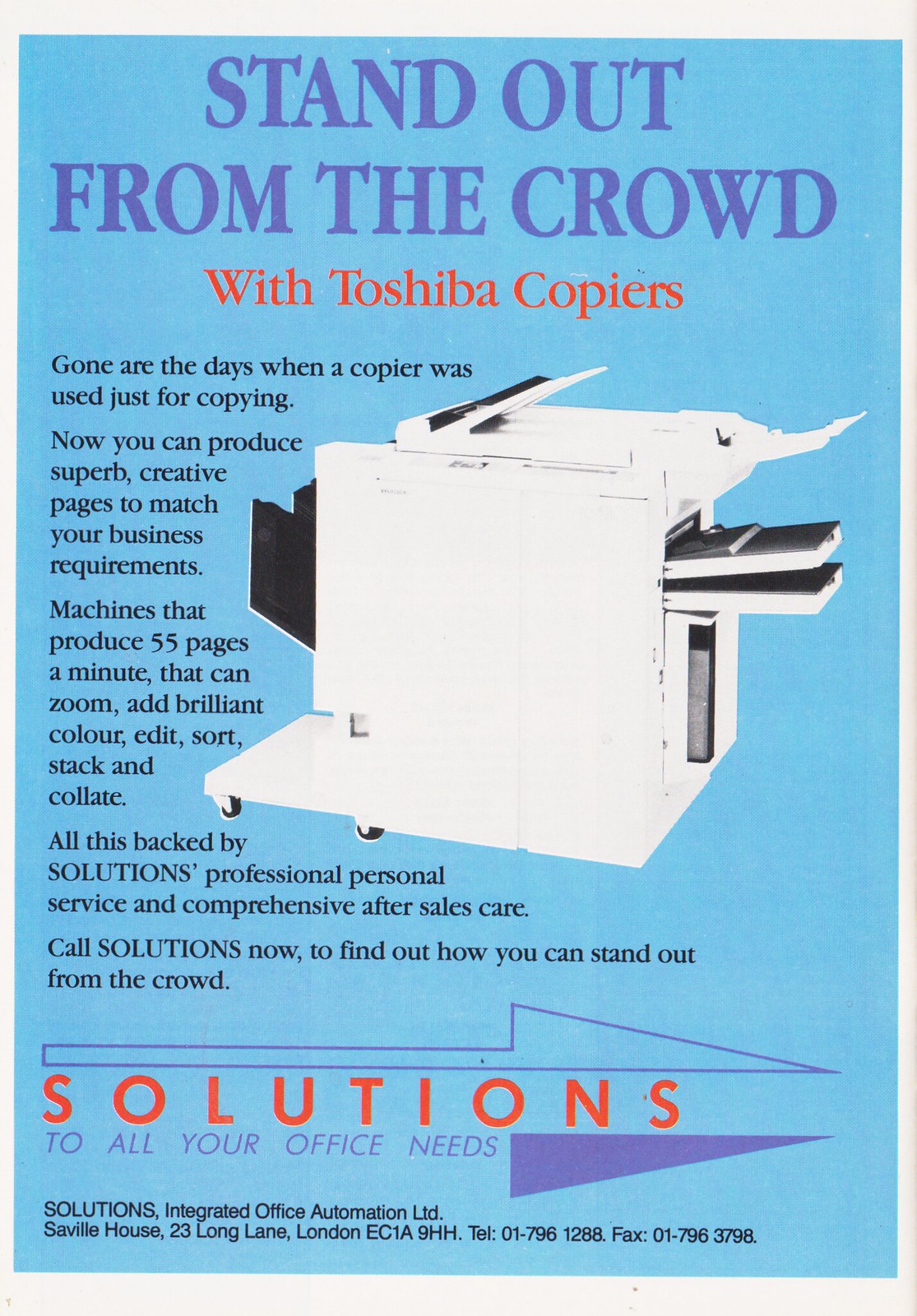This is an advertisement for Toshiba copiers, likely from the late 1980s or early 1990s. The ad features a vibrant blue background with a mix of purple and red text, showcasing a gleaming white photocopier slightly right of center. The prominent headline reads, "Stand out from the crowd with Toshiba copiers," emphasizing the machine's ability to produce high-quality, creative pages tailored to business needs. Beneath, it declares, "Gone are the days when a copier was just used for copying," highlighting advanced features such as producing 55 pages per minute, zoom, brilliant color, editing, sorting, stacking, and collating. The ad concludes with, "Solutions to all your office needs," and includes an address at the bottom, indicating it was printed in London by Solutions Integrated Office Automation, LTD.